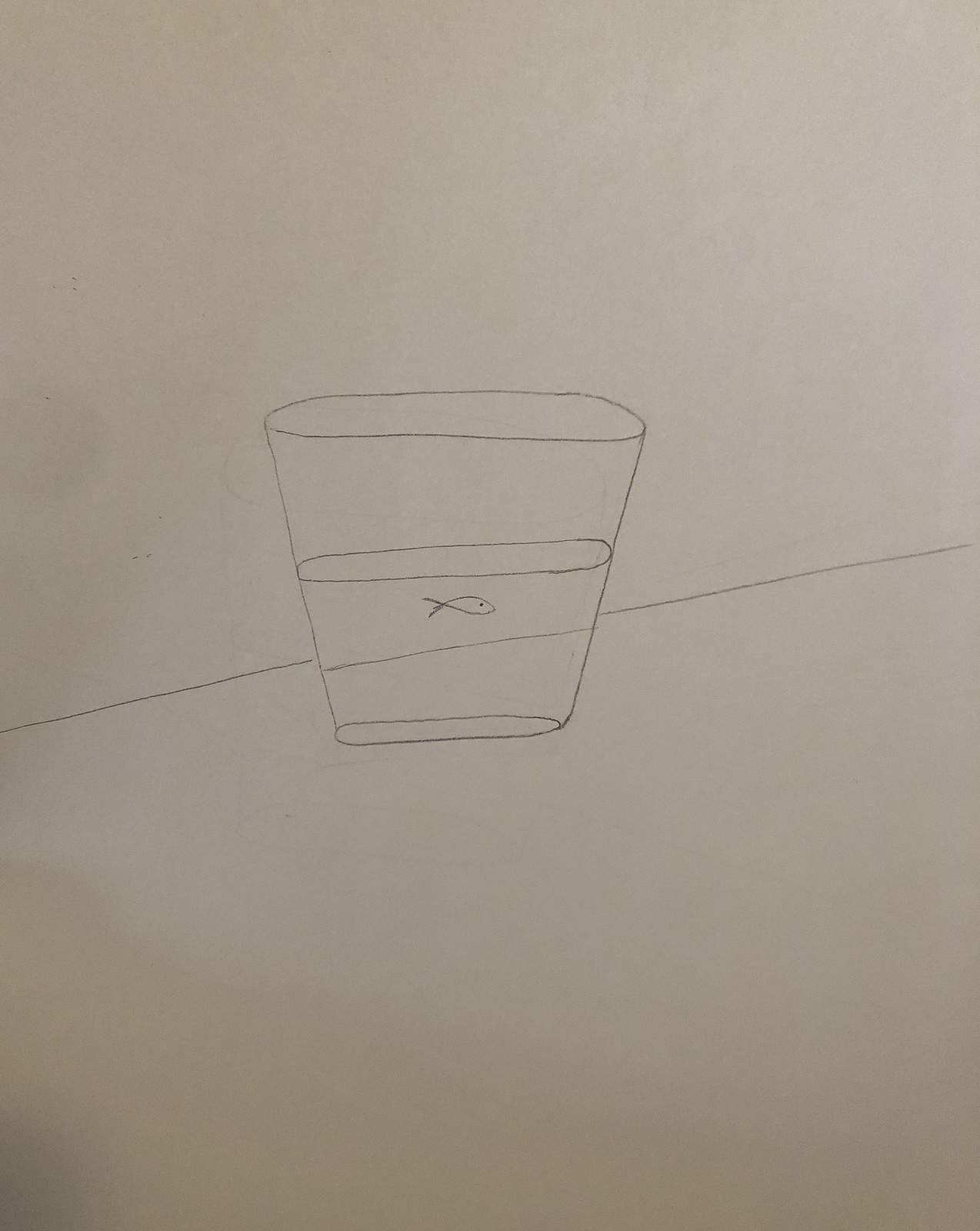A simple pencil drawing depicts a fish in a short, transparent cup, positioned on what appears to be a countertop. The fish, drawn with a crisscross pattern for its body and a distinct eyeball, is facing to the right. The background is a slightly darkened white piece of paper, adding subtle texture to the scene. A horizontal line runs behind the cup, suggesting the edge of the countertop. The minimalist style and absence of color highlight the intricacy of the pencil work and the clear visibility of the fish within the water of the cup.